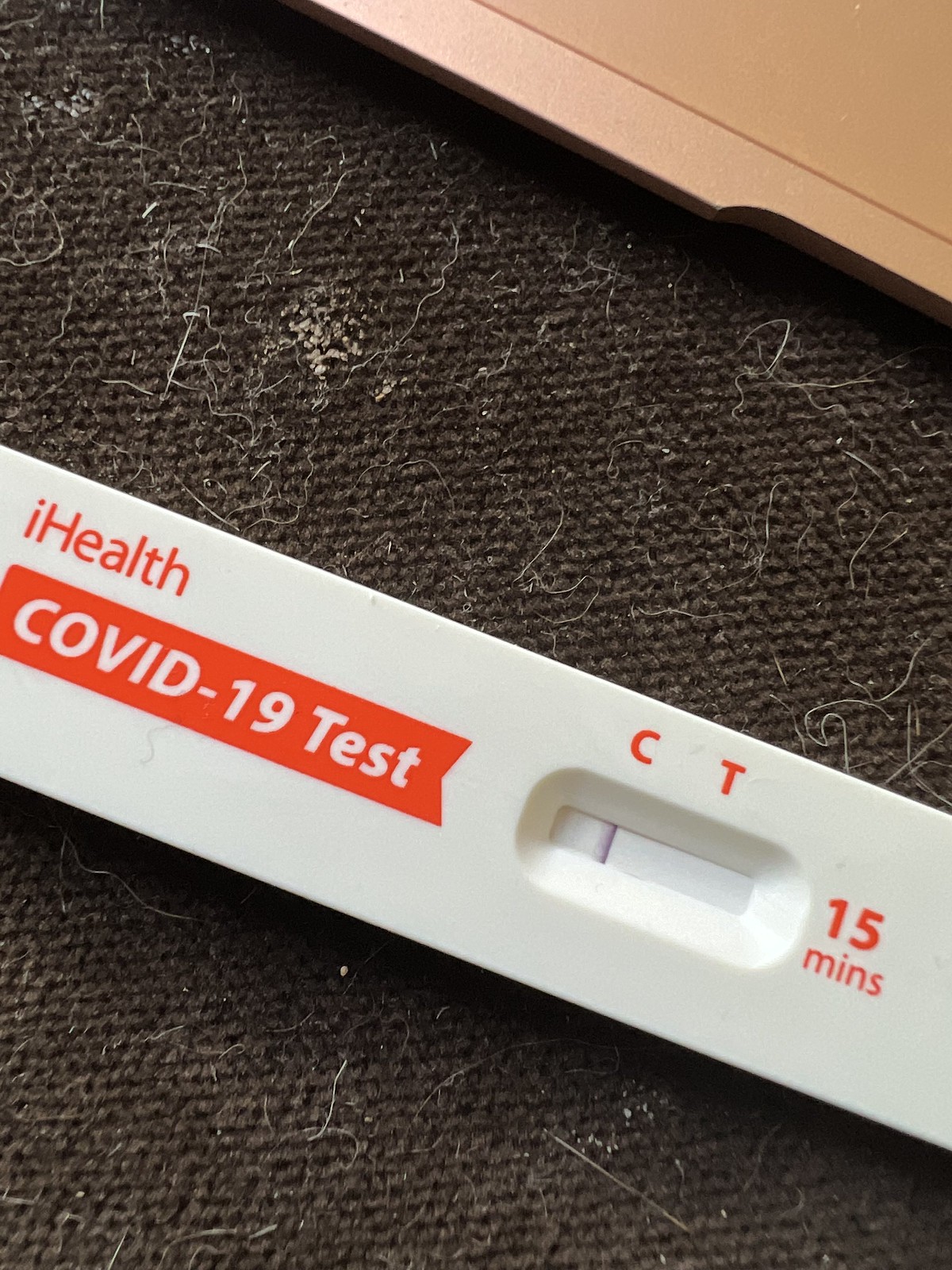A single COVID-19 test lies on a black, slightly dirty surface covered with white fur. The test, marked with "iHealth" in capitalized letters and an orange "COVID-19 Test" label, features a long, round window with one dark purplish line trending towards the left side. Above the window, the letters "C" and "T" are visible in orange, alongside the number "15 mins." The white test kit stands out against an orange background, prominently displaying the brand and test name in a clear, organized manner. In the upper section of the image, there is a brown object, possibly part of a table, whose exact nature remains indeterminate.